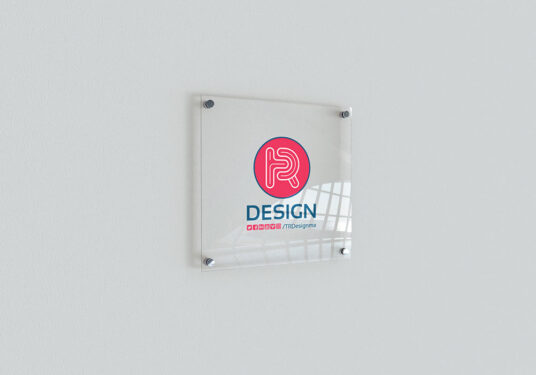This photograph features a clear plastic sign or plaque securely fastened to a white or light gray wall with silver screws at each corner. Central to the plaque is a distinctive red circular logo with a decorative, somewhat abstract white 'R' inside, bordered by a thin blue outline. Below the logo, the word "DESIGN" is prominently displayed in blue capital letters. Further beneath, there's additional text in red and blue, likely referencing "TR designs MA" or similar, though it's too small to read clearly. The plaque has a reflective quality, hinting at a large window somewhere in the vicinity.